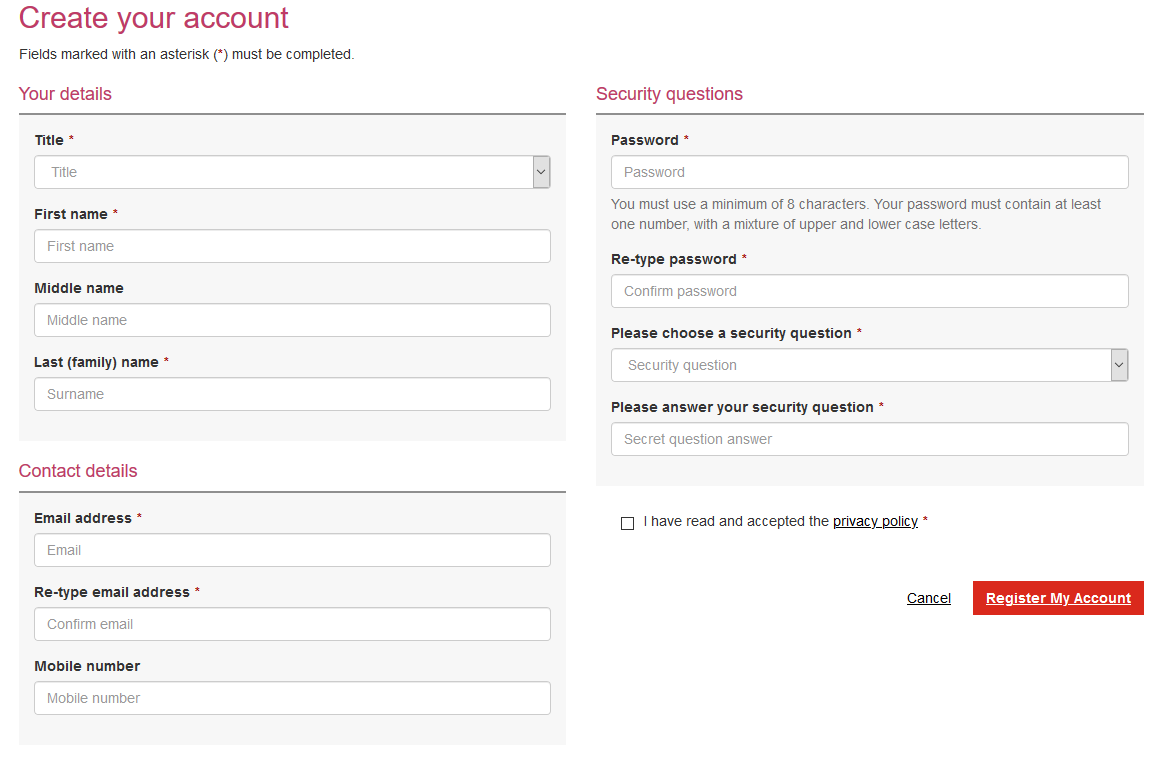The image depicts a user registration form with sections marked in red for emphasis. In the upper left corner, the heading "Create Your Account" is highlighted in red. Below this, a note clarifies that fields marked with a small red asterisk (*) must be completed.

Under the "Your Details" section, also in red, are fields requiring the user's title, first name, last family name, and optionally, the middle name—all marked with a red asterisk to indicate mandatory input.

To the right, the "Security Questions" section in red prompts users to create a password, retype the password, choose a security question, and provide an answer to the security question, with each field indicated as mandatory by a red asterisk.

Below, there's a checkbox accompanied by the text "I have read and accepted the Privacy Policy," with "Privacy Policy" underlined, suggesting a hyperlink. Further down, the word "Cancel" is underlined, indicating it may be a clickable option, while the button "Register My Account" is displayed in white text inside a prominent red box.

On the left, the "Contact Details" section in red includes fields for "Email Address" and "Retype Email Address," each with a red asterisk. The section concludes with a field for "Mobile Number," accompanied by a long rectangle input box for entering the number.